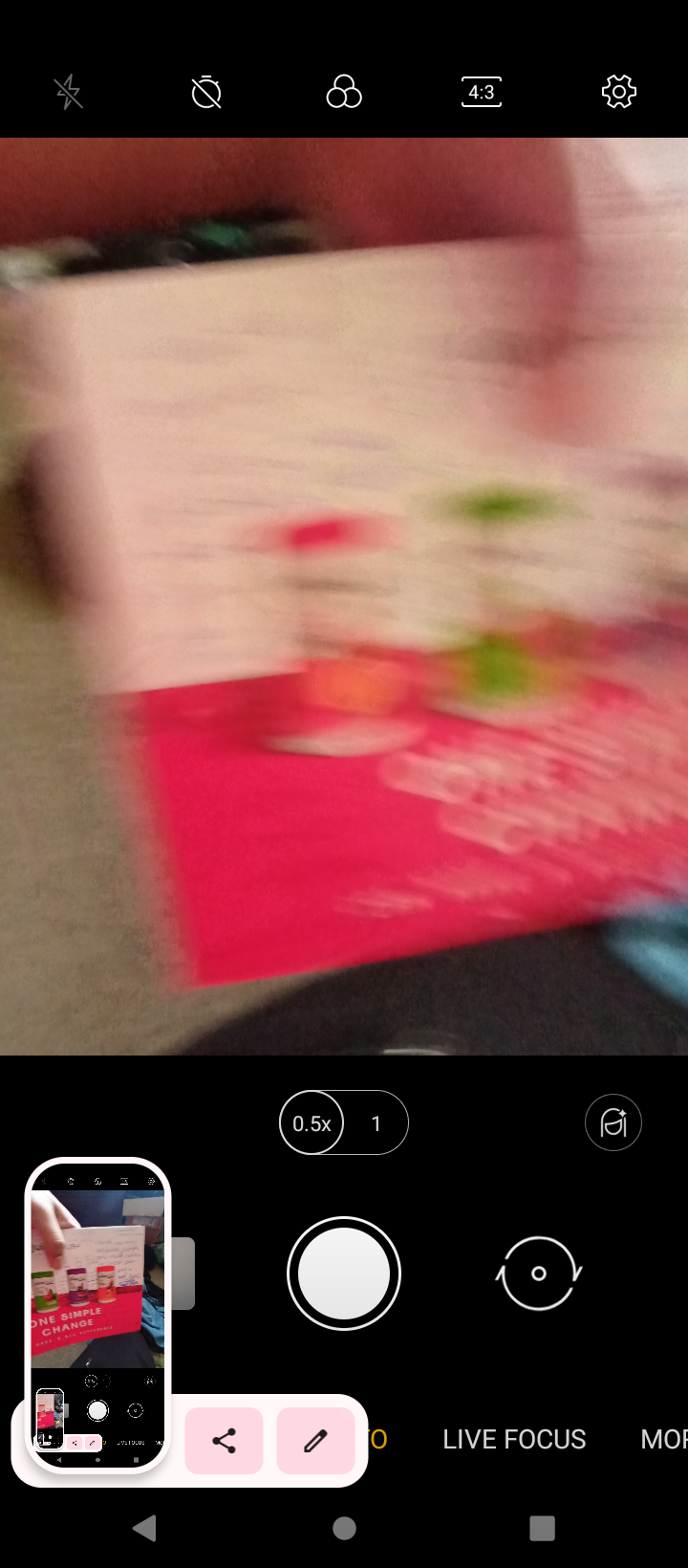The image is a very blurry screen capture taken inside a cell phone's camera app. At the top of the screen, there is a black ribbon displaying various cell phone icons, including indicators for flash and timer settings, with the aspect ratio set to 4:3. The main section of the image is dominated by a highly blurred view of what seems to be a person's hand holding a flyer. This flyer appears to advertise three small containers, potentially varieties of yogurt, in red/orange, green, and purple colors. The flyer includes some text, partially readable as "1 CHAK". At the bottom of the screen, the camera app controls are visible, including buttons for Share, Edit, Live Focus, and More, along with standard navigation buttons like a back arrow, a round shutter button, and a square symbol. Additionally, there is an inset overlay at the bottom corner showing a clearer, unblurred version of the flyer image, which confirms the three containers depicted in the main blurry image.